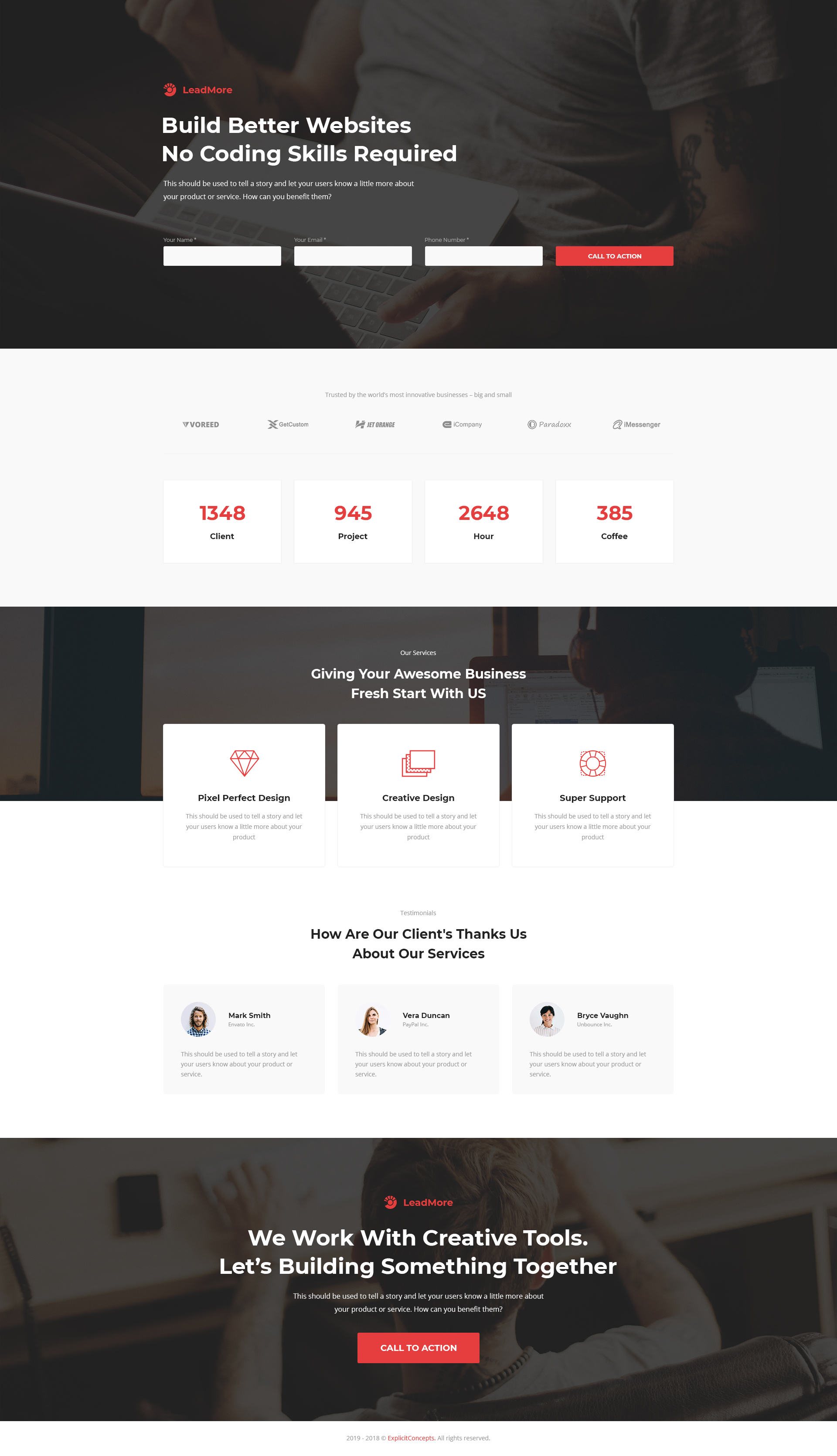**Caption:**

The image depicts a desktop website's landing page, though the web address, specific browser, and operating system are not visible. Prominently featured at the top is a red circle encircled by a red semi-circle, with bold white text proclaiming “Lead More, Build Better Websites - No Coding Skills Required.” This section urges users to recognize the benefits of the product or service offered, emphasizing storytelling. Beneath this slogan, forms exist for entering a name, email, and phone number, all mandatory fields. A red call-to-action button with white text is situated near these input fields.

The background shows a tattooed, white man in a white shirt holding a laptop, with one clenched fist, creating a dynamic and motivational visual. Below this image, the text reads, “Trusted by the world’s most innovative businesses, big and small,” listing companies such as Voreed, Get Custom, Set, Orange, iCompany, Paradox, and iMessenger—names possibly fictitious or obscure.

Red-highlighted statistics provide insight into the business's impact: 1,348 clients, 945 projects, 2,648 hours of work, and 385 coffees consumed.

Further down, a section labeled “Our Services” describes the company’s offerings with slogans like “Giving your awesome business a fresh start with us.” Service highlights include a red diamond labeled “Pixel Perfect Design,” “Creative Design” indicated by red pieces of paper, and “Super Support” represented by a life raft image. Each offering repeats a message about storytelling and user engagement.

The testimonial section features three clients: Mark Smith from Envato Inc., Vera Duncan from PayPal Inc., and Bryce Vaughn from Unbounce Inc. All of whom share identical feedback phrasing: “This should be used to tell a story and let your users know about your product or service.”

Further down, text appears again: “Lead More – We work with creative tools. Let's build something together,” albeit with grammatical issues: "Let's building something together." Below is another red call-to-action box, situated next to the image of a person in a white shirt sitting in a chair, possibly at a desk, using a desktop with a phone alongside.

At the very bottom, despite the logical inconsistency in years, the footer reads “2019 to 2018 Explicit Concepts. All rights reserved,” suggesting this might be an unfinished or sample website.